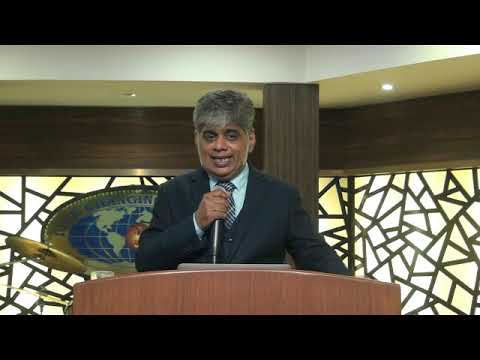A man with gray, fluffy hair and dark skin stands confidently at a wooden podium, speaking into a black microphone he holds in his hand. He is dressed in a navy blue suit jacket over a light blue dress shirt, complemented by a black and white tie. Behind him, a backdrop of striking yellow glass windows with intricate geometric patterns framed by golden lines illuminates the scene. These windows depict various triangular and trapezoidal shapes, adding a warm glow to the setting. A large globe emblem, rendered in gold and blue, prominently decorates the space behind him. To his side, a drum kit is partially visible, marked by the distinctive top hat cymbal. The overall setting suggests this is a modern-day church, as wooden pillars and panels frame the scene, and there is a framed sign mentioning "church" in the background, implying that the man may be delivering a sermon or leading a meeting as a pastor.